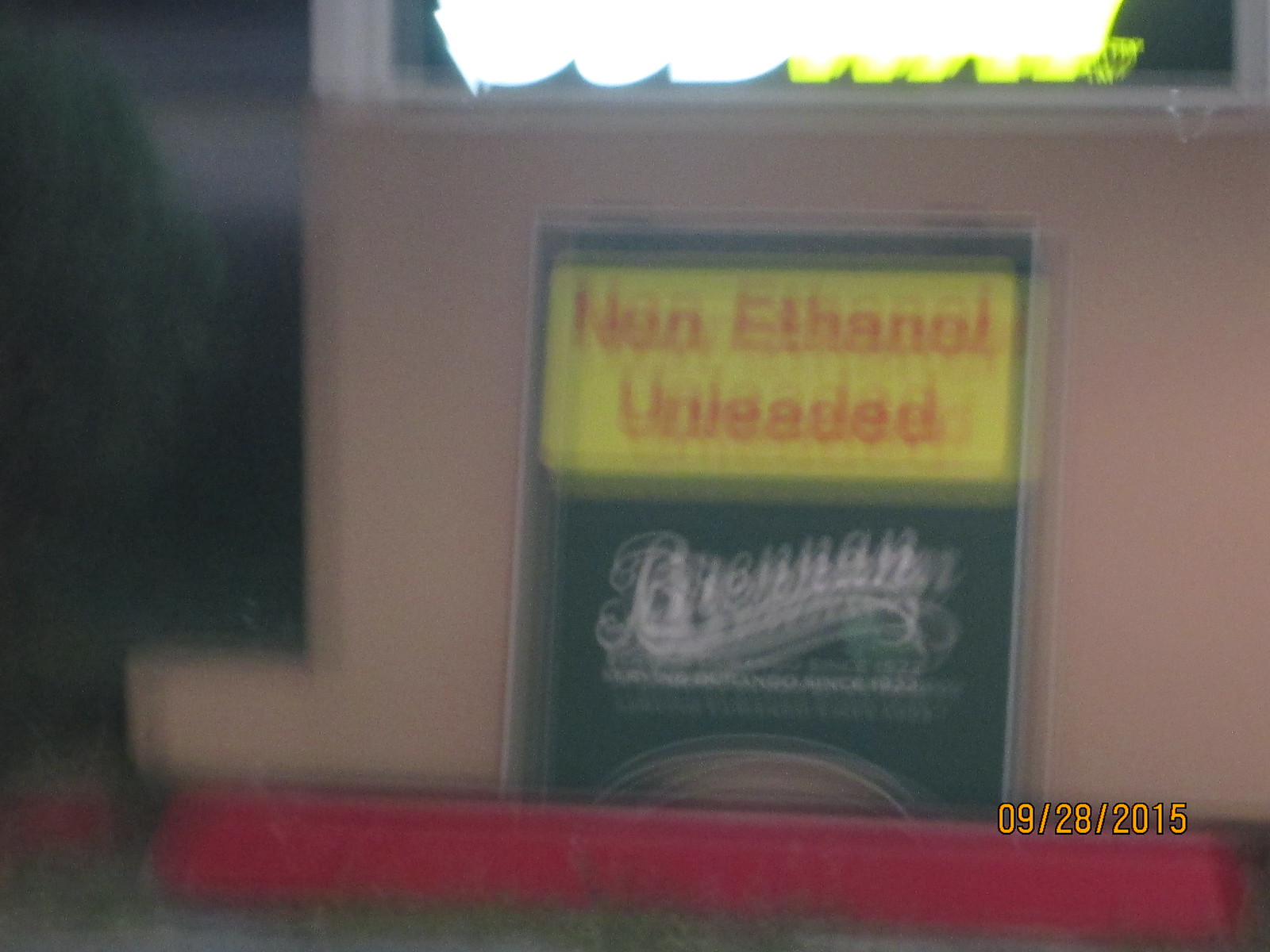In this blurry image, we see a gas station scene. The focal point is a green sign with a yellow inset section, prominently featuring red lettering that reads "Non-Ethanol Unleaded." Though the lower part of the sign is less clear, it appears to say "Brennan's." The sign is propped against a beige exterior wall, which also includes a window positioned above the sign. In front of this setup, there is a red raised platform designed for cars to park. The overall setting is somewhat indistinct due to the image's blurriness, but these elements combine to convey a familiar but slightly vague roadside moment.